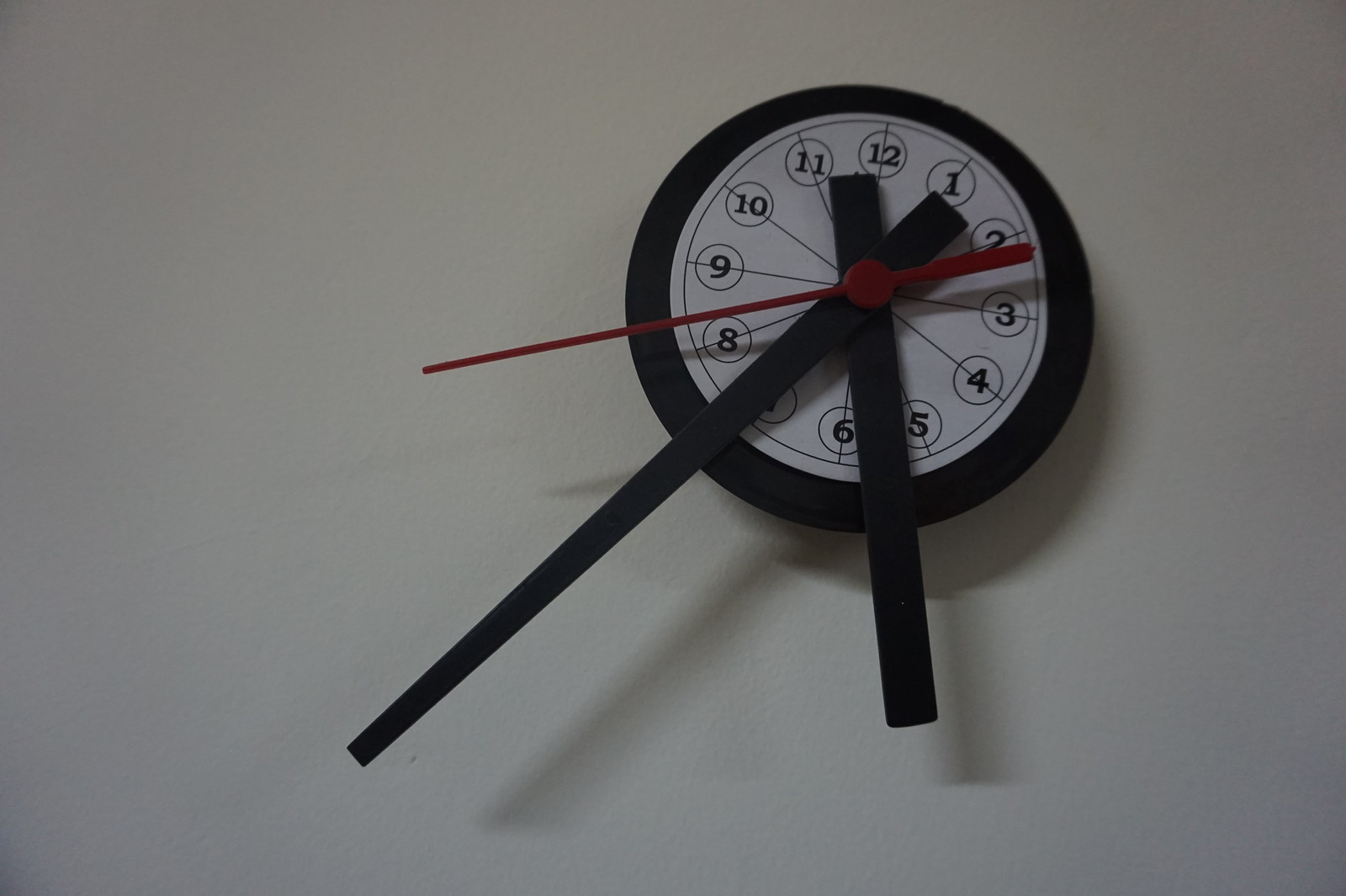This photograph features a meticulously detailed miniature toy clock resting on a pristine white surface. The clock boasts a clean, white face accentuated with bold black numerals and black circles that frame each number. These elements are seamlessly integrated into a circular fashion, dividing the clock into well-defined sections with subtle lines. The clock has two strikingly long black hands, which extend beyond the clock face and drape over the edge of the white surface, adding a whimsical touch. A vibrant red second hand adds a pop of color to the composition. The clock's body is sleek and black, creating a striking contrast against its white face and the surface it rests upon. The excellent image quality features no blurriness or distortion, making every detail of the clock and its soft shadow on the table crystal clear. This captivating image captures the charm and precision of the miniature clock with remarkable clarity and finesse.